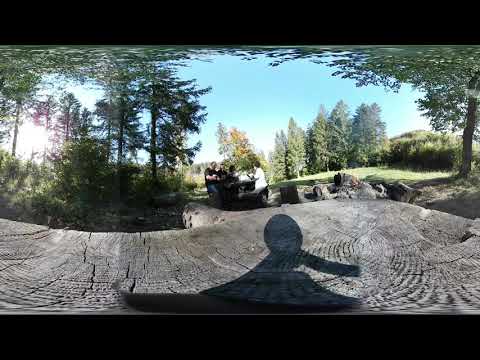This outdoor photo, taken in a park, captures a scene dominated by nature and social interaction. The image is vertical and rectangular with horizontal black stripes framing the top and bottom. In the foreground, just below the center, there's a large cut log, its intricate rings visible in the gray wood. This log sits on a flat, stone-tiled patio area that casts a shadow from the bright sun, hinting at the clear, cloudless blue sky above.

The scene appears to be viewed from a slightly elevated position, looking down into a lush, green park. To the left and right, tall evergreen trees form a dense, verdant canopy, their leaves touching the edges of the frame and creating a natural border.

At the heart of the photo, a group of several people—mostly men—are gathered, possibly seated around a bench. The figures are somewhat blurry, but distinguishable details suggest that one person on the far left is wearing a black short-sleeved shirt, while another on the far right dons a white shirt. They are surrounded by the tranquil greenery of the park, with a wide, grassy area extending to the right.

The overall atmosphere conveyed by the image is one of serene, natural beauty on a bright, sunny day, making it a picturesque snapshot of a peaceful outdoor gathering.